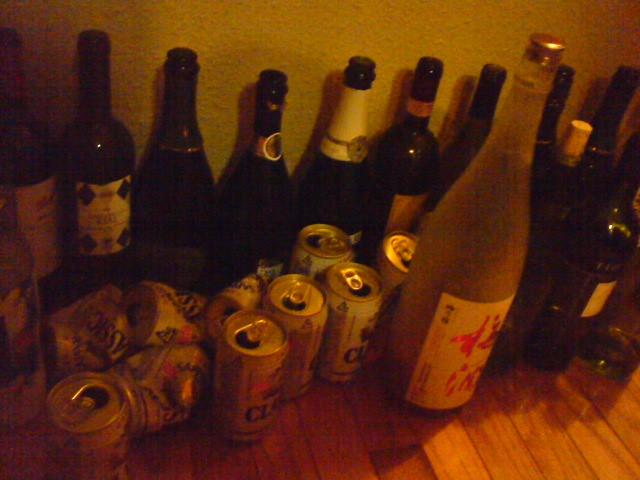The photograph showcases an indoor scene featuring a collection of various empty bottles and cans prominently displayed on a hardwood floor, which appears to be red oak or perhaps two-inch fir flooring. Against a predominantly white or yellow, possibly green, wall, there is a back row filled with numerous wine bottles, mostly dark in color, some adorned with labels or stickers. In front of the wine bottles, there are about ten aluminum beer cans; half of these cans are crushed while the others remain intact. The majority of bottles are brown and include both beer and wine varieties, with a few clear bottles among them. Of particular note is a clear bottle with a brass or gold lid and a white label featuring red text that appears Japanese. One of the wine bottles in the front row features a cork. This detailed arrangement of empty bottles and cans, possibly the aftermath of a gathering, rests haphazardly on the wooden floor.